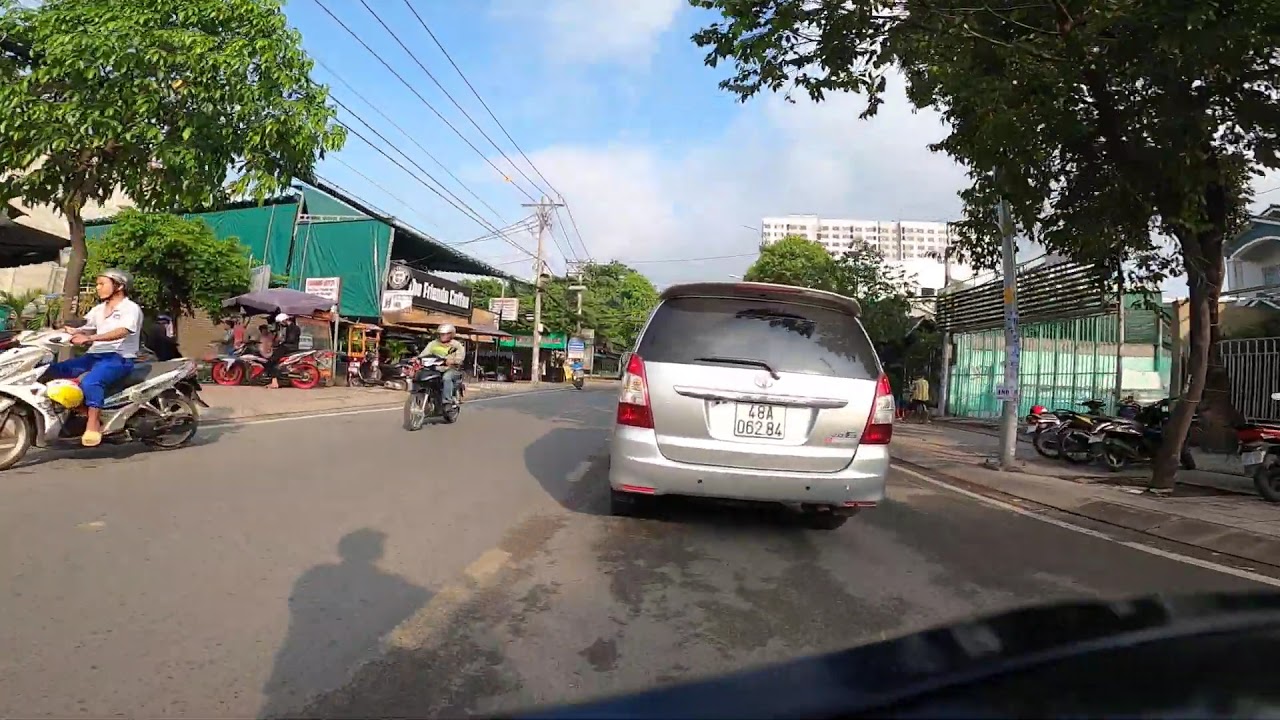This photograph captures a bustling street scene from the perspective of someone inside a car, visible in the bottom right corner of the image. The day is partly cloudy, with the sun off to the right casting shadows, including that of a cyclist who remains out of sight. Directly ahead is a gray minivan with a foreign license plate. To the right of the minivan, a sidewalk with a tree and a row of parked scooters can be seen. Across the road, a trio of motorcyclists is spread out along the left lane, with one near the car, one further down, and a third barely visible in the distance.

Shops and possibly market stalls line both sides of this narrow, somewhat rundown street, suggesting the setting might be a less developed area, potentially in a foreign country. The scene includes green trees, grey buildings, and multiple power lines. A large white building dominates the background, beneath a sky filled with clouds. The lower half of the image is primarily the street, characterized by its weathered surface, while the sides are framed by sidewalks, greenery, and commercial structures, creating a colorful mix of grey, blue, and green tones throughout the photograph.